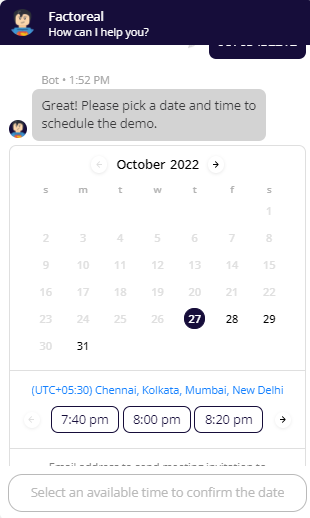A detailed screenshot of a web chat interface with an AI assistant is displayed. The interface features a blue header at the top, with a profile picture of an animated Superman on the far left side. This profile image, rendered in an animation style, sits next to the name of the AI or the company, "Factor Reel," which is accompanied by a small white text below that reads, "How can I help you?"

The main body of the chat, which has a white background, showcases the initial message from the AI. The message header, marked with the label "Bot" and a timestamp, introduces a gray message bubble containing the text: "Great, please pick a time and date to schedule the demo." Following this message, a pop-up box featuring a calendar appears, allowing the user to select their preferred date.

Beneath the calendar, a series of time slots are displayed in clickable boxes, with three specific times shown initially. An arrow to the right indicates that additional times can be accessed through scrolling. Above these time slots, there is a blue hyperlinked text for time zone settings, which specifies that the listed times are in New Delhi time.